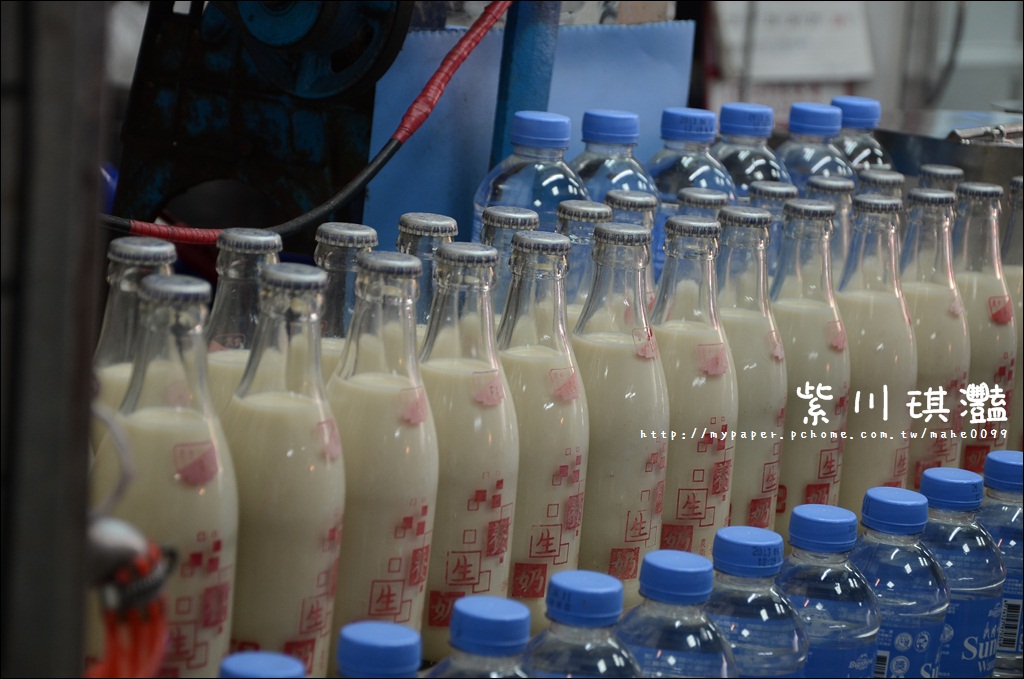This photograph depicts an assembly line in a Taiwanese beverage factory, as indicated by the text "http http://mypaper.pchome.com.tw http://mypaper.phome.com.tw" displayed prominently in the center right. The image showcases a three-tiered shelving system. The bottom shelf is lined with plastic bottles capped in blue, filled with clear water. The middle shelf features two rows: the front row consists of glass milk bottles with pop-off metal tops and pink writing, while the back row mirrors the bottom shelf with more water bottles. The top shelf remains out of the frame. Visible wires and machinery elements hint at the industrial setting. The Asian text on the image further suggests its Taiwanese origin.